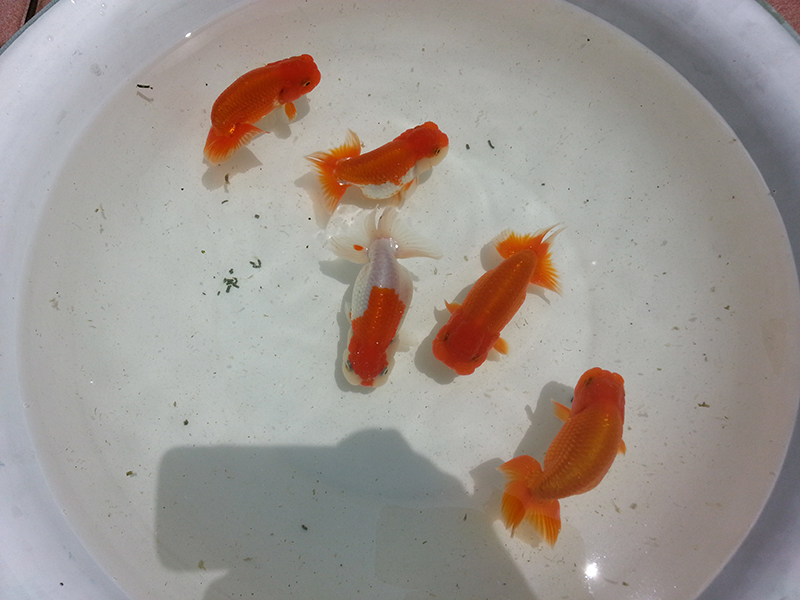In the photograph, five koi fish, resembling goldfish with their distinct bodies, are swimming in a shallow pool of water within a wide, white ceramic bowl. The bowl's rim is highlighted with a greenish hue and features speckles of pink and pastel colors, adding a decorative touch. The koi are primarily bright orange, evocative of classic goldfish, with three displaying a consistent gold color. The other two have noticeable patches of white, creating a striking contrast. Positioned in various directions, these fish appear in slightly cloudy water, marred by tiny bits of floating debris. A shadow, presumably of the person taking the photo, casts a soft silhouette over the scene, adding a candid dimension to this unusual display of aquatic life in a dinnerware vessel.